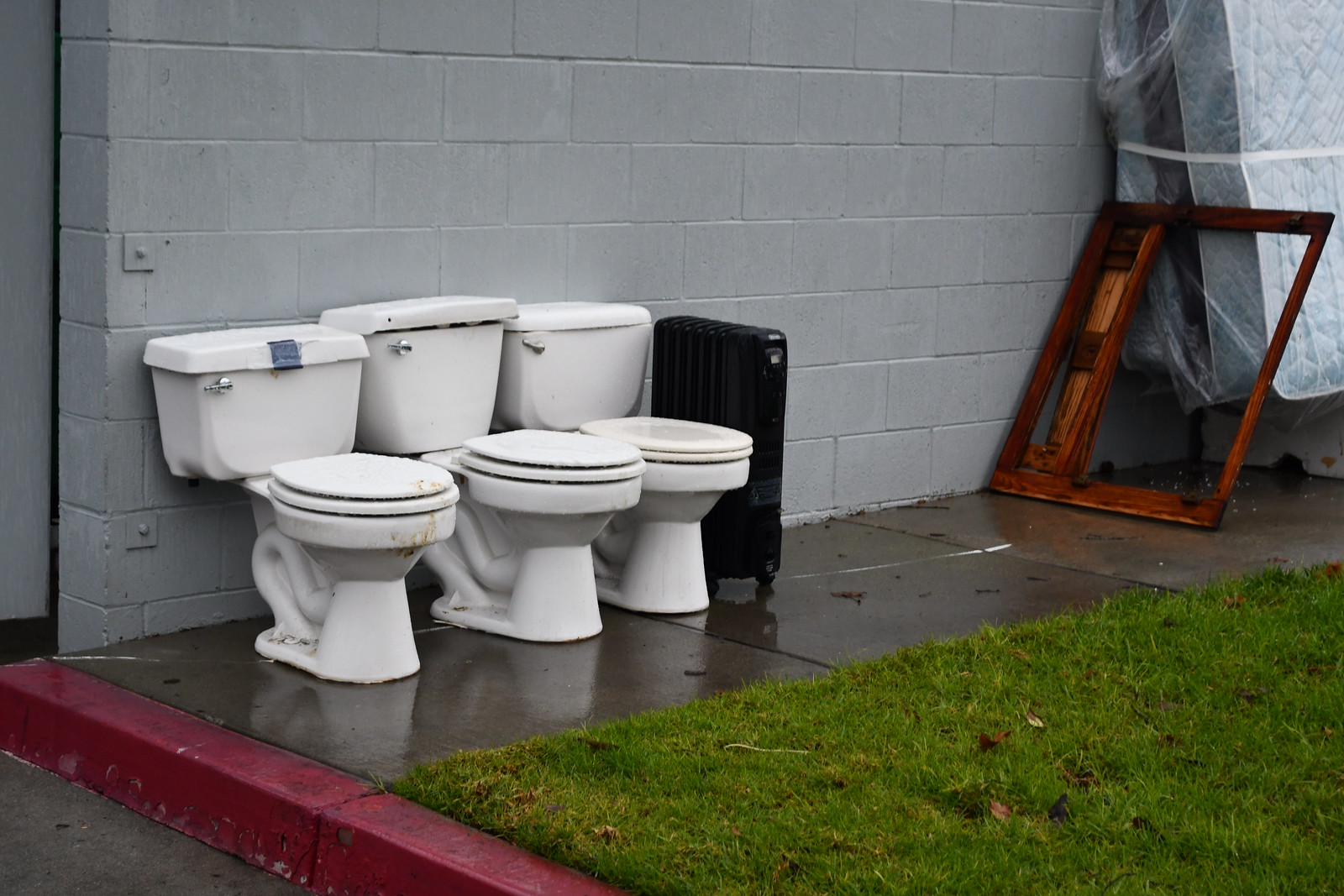The image depicts a row of three toilets lined up against a large, blue-grey brick wall outside, on what seems to be a slightly wet, cement sidewalk. The sidewalk transitions into a red-painted curb on the bottom left and a patch of very green grass on the bottom right. Each toilet, identical in size and height, has a stainless steel lever for flushing and looks quite dirty, with brown stains visible on the one on the left and a piece of tape on the lid of another. To the right of the toilets, there is a black oil-thin radiator heater and several mattresses wrapped in plastic, leaning up against the wall. Nearby, a discarded wooden cabinet frame rests against the mattress stack, adding to the scene of abandonment and disarray.